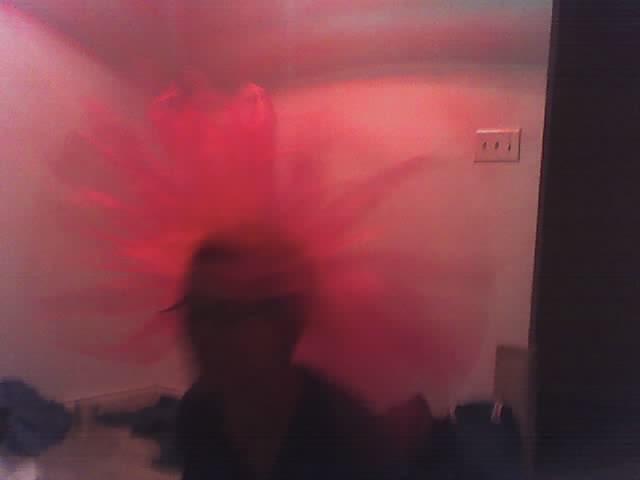This blurry digital photo, taken indoors, features a white-walled room with white baseboards and a light switch panel with three switches—two up and one down. The switch cover is white and is located on the left side of the image near where a black door frame possibly leading to a darkened area or hallway stands. Central to the image is a young person, possibly around 13 years old, of indeterminate gender. They have short dark hair and are wearing a black or v-neck shirt, which is partly obscured by blurriness. A distinctive pink cloud or halo effect encircles their head; this could be caused by twirling dreadlocks, a mohawk, a tutu, or even a burst of pink dust. The face is not visible due to the blurriness, but the person might be wearing glasses. There appears to be clothing strewn on the floor, and the overall chaotic yet captivating vibe of the image draws attention to the mysterious and dynamic blur around the person's head.